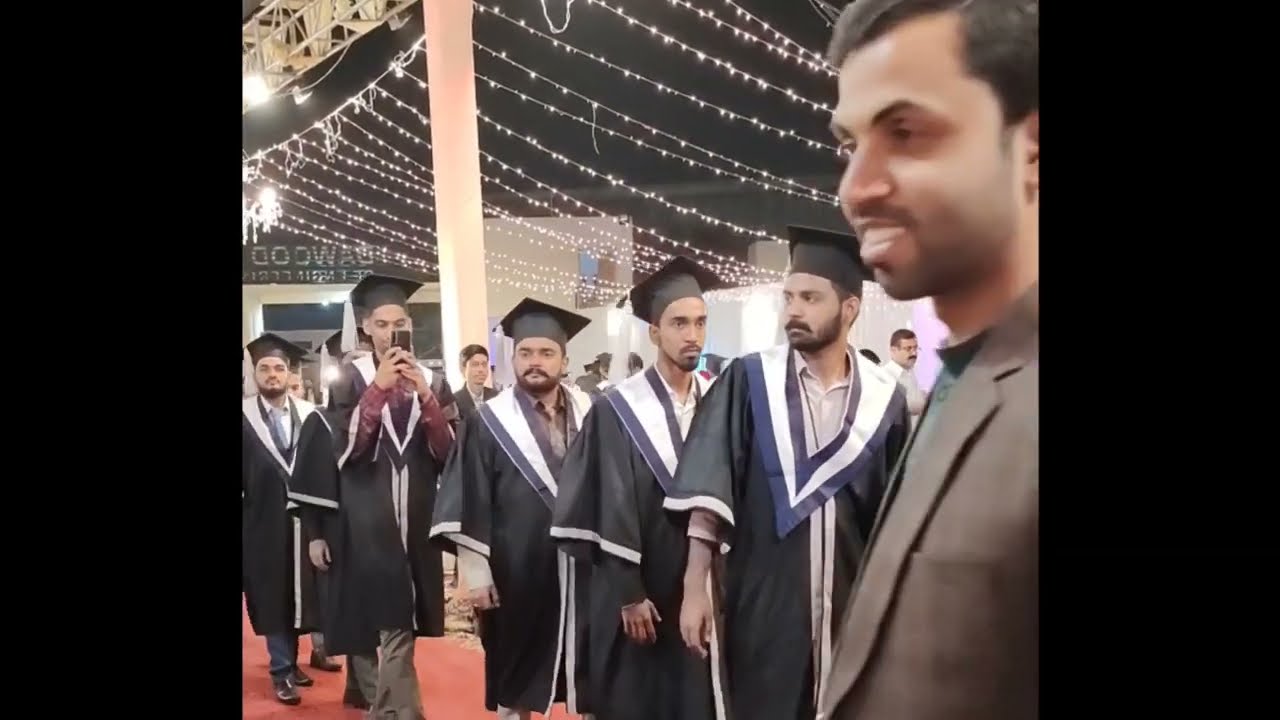The image depicts a vibrant graduation ceremony, likely set in an auditorium adorned with string lights that illuminate the festive atmosphere. Dominating the foreground is a man in a beige overcoat with a high-collared shirt, inadvertently captured mid-walk and smiling warmly. The central area is bustling with activity where a line of graduates, dressed in black gowns with navy collars trimmed in white, marches towards a stage. The gowns feature white-striped sleeves, and most graduates don black caps, highlighting the formal occasion. Among the six men in this line, one is seen holding a cell phone, possibly snapping a memory.

The background is animated with people mingling, capturing moments on their cell phones, against a backdrop featuring cut-out cityscape windows and intriguing lit-up letters that read "God, Wow" or "Goo Wow". The celebratory mood is palpable with graduates of apparent Middle Eastern descent, suggesting a diverse and inclusive event. The setting is further enriched by a red carpet and white-walled interior, completing the snapshot of an enthusiastic and memorable graduation ceremony.